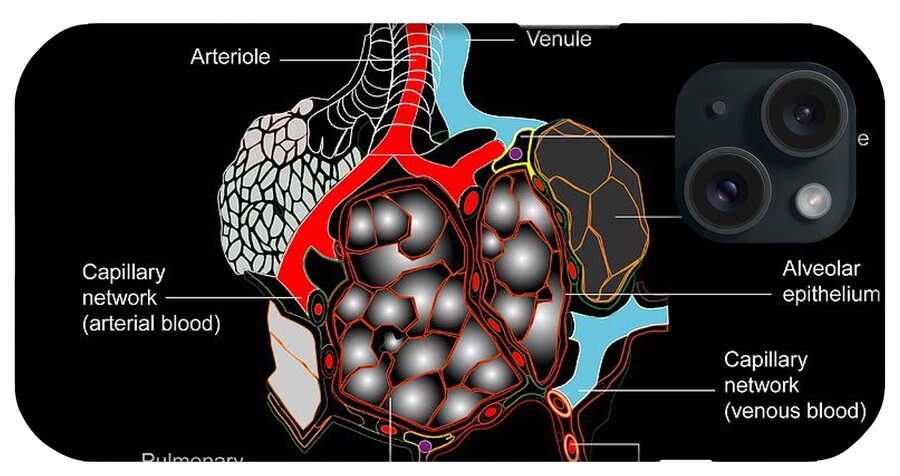The image is a horizontally oriented, abstract scientific illustration of human anatomy, specifically the respiratory and circulatory systems. Set against a black background that contrasts sharply with the colorful elements of the diagram, it appears to be printed on the back case of a smartphone. The central graphic prominently features stylized lungs with interconnected red (arterial blood) and blue (venous blood) veins. Key anatomical labels include "alveolar epithelium" on the right side, "capillary network, venous blood" at the bottom right, and "capillary network, arterial blood" on the left. The top of the illustration indicates "arterial" linked to the largest red vein and "venial" to the large blue vein. In the upper right corner, there is an inset resembling a camera or webcam with two lenses, which partly obscures some of the white text behind it. A small dot or speaker appears at the top left, and a light on the bottom right of this inset, with an "E" behind it, implies technological integration or a potential biotechnical application. The fragmented bottom part of the diagram teases the word "pulmonary" with an arrow pointing upwards. Overall, this detailed and visually striking illustration seems to function as both an educational tool and a decorative element on a tech device.